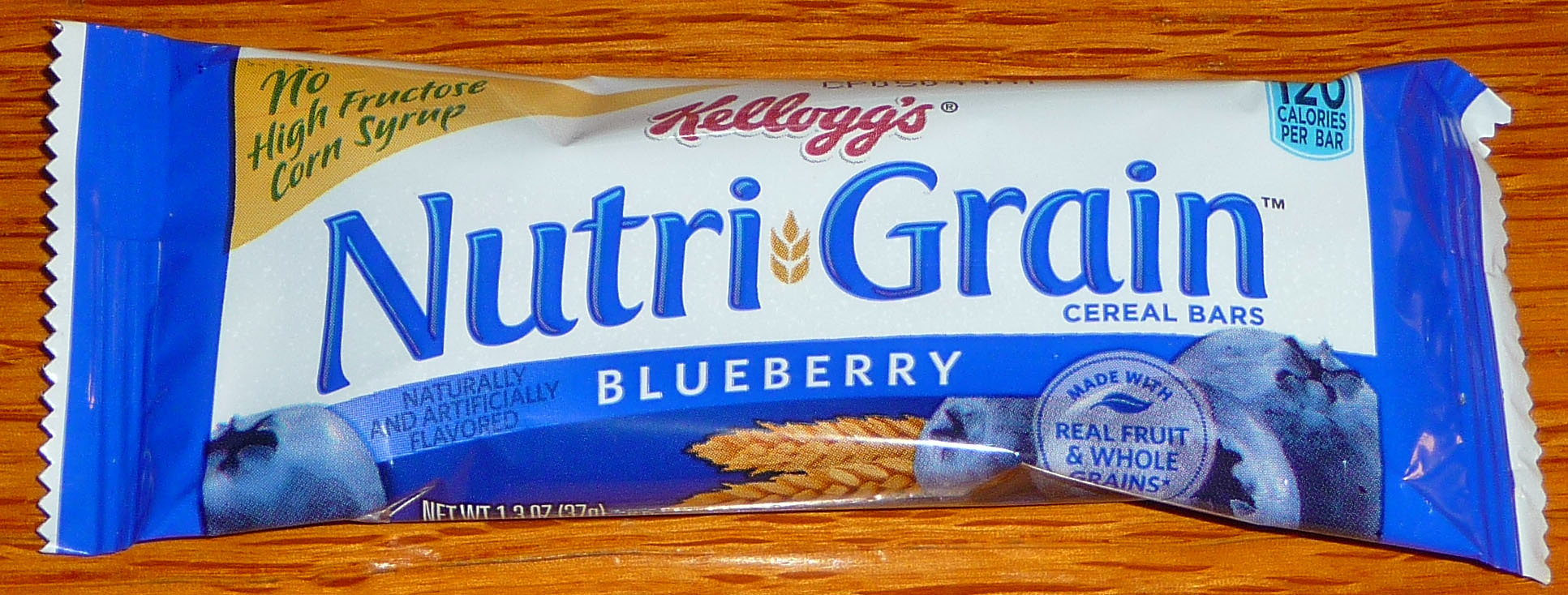A meticulously arranged photograph showcases a single Nutri-Grain bar elegantly positioned atop a light wood-colored countertop, exuding a rustic yet inviting aesthetic. The Nutri-Grain bar is encased in a distinctive blue and white package. At the top of the package, the iconic brand name "Kellogg's" is prominently displayed in elegant red cursive lettering. Directly beneath, the product name "Nutri-Grain" is featured in bold blue text. Below this, in a crisp white font, the flavor "Blueberry" is clearly indicated. The packaging is further adorned with vibrant images of juicy blueberries along the sides, enhancing its appeal. In the top corner, a reassuring label proudly states "No High Fructose Corn Syrup," while the bottom corner highlights the product's wholesome credentials with the phrase "Made with Real Fruit and Whole Grains." This detailed and descriptive image captures the essence of a convenient, nutritious snack option.